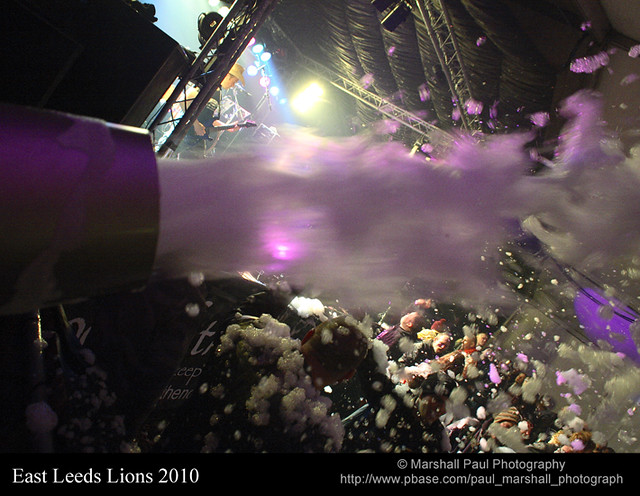The photograph captures an energetic moment at a live concert, possibly taken indoors, emphasizing the vibrant atmosphere and dynamic elements of the scene. The band onstage is illuminated by bright spotlights in hues of blue, green, and red, cutting through the dimly lit environment. In the forefront, a guitarist is visible, distinguished by his tan cowboy hat, black t-shirt with a white logo, and black guitar. A striking feature of the image is a purple cannon on the left, actively shooting light purple foam or suds out towards the tightly packed crowd below. The foam creates a whimsical, almost surreal visual, reminiscent of scenes from "Willy Wonka," enveloping the audience and slightly obscuring the stage. Despite this, the stage’s backdrop of blue lights and what appear to be black coverings, akin to garbage bags, can be discerned. The photograph includes footer text, with "East Leeds Lions 2010" positioned in white print on the lower left and a copyright notice, "Copyright Marshall Paul Photography" along with a web address on the lower right.